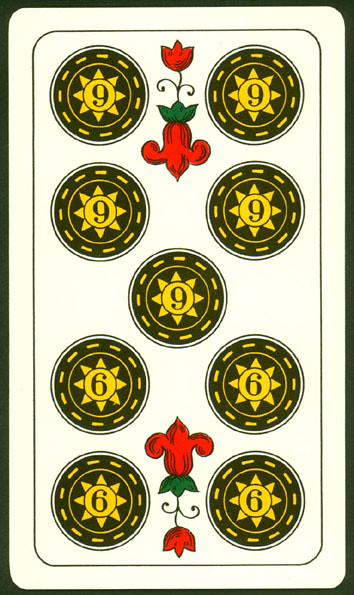Close-up photograph of a playing card featuring the Nine of Spades. The card is oriented number side up, displaying a symmetrical arrangement of nine black spade symbols, each contained within a circular pattern. 

The card is divided into three main sections:
- **Upper Section:** Four spade symbols are positioned in a grid of two rows and two columns.
- **Central Section:** One spade symbol is centered between the top and bottom sections.
- **Lower Section:** A mirror image of the upper section with four spade symbols arranged similarly.

Each spade symbol is encapsulated in a decorative circular pattern. Each circle features a yellow center, a broken outer ring, and two numbers—nine above and six below—with black numerals. The circles are surrounded by an outer white ring. 

Interspersed between these symmetrical patterns, a simple red floral drawing resembling a spade with leaves and a blooming flower decorates the top, center, and bottom sections of the card. 

The entire card is bounded by an outer black rectangle with smooth corners, giving it a finished look. Notably, the card features no additional text, words, or print, focusing purely on the design elements.